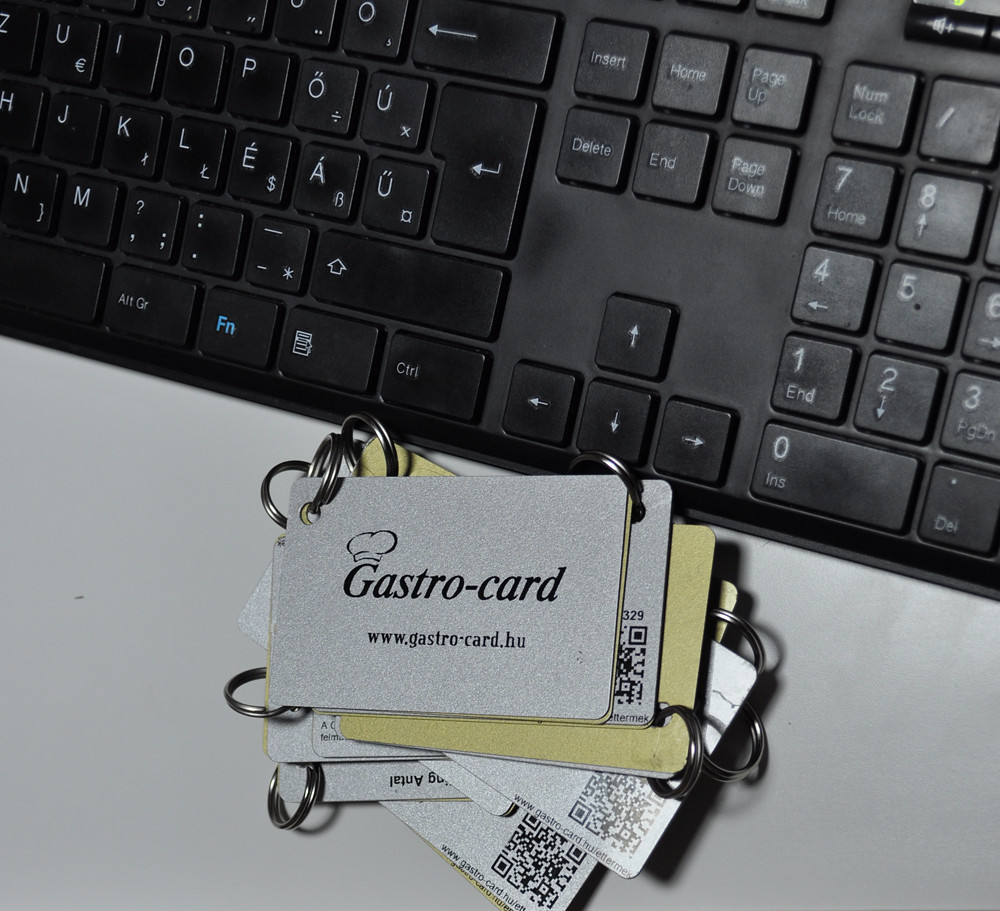The image showcases a close-up of a well-used, black computer keyboard, prominently displaying its partially visible European layout with its number pad on the right and half of the letters on the left. The keyboard, which appears a bit dirty and aged, rests on a gray surface. In the foreground, there is a stack of swipe cards, some facing up and others down, with keychain rings through holes punched in their top left corners. The cards, primarily white and yellow in color, bear the inscription "GASTROCARD" in black lettering, accompanied by the website address "www.gastrocard.hu" underneath. Notably, the 'G' in "GASTROCARD" is adorned with a chef's hat logo, emphasizing a culinary theme.